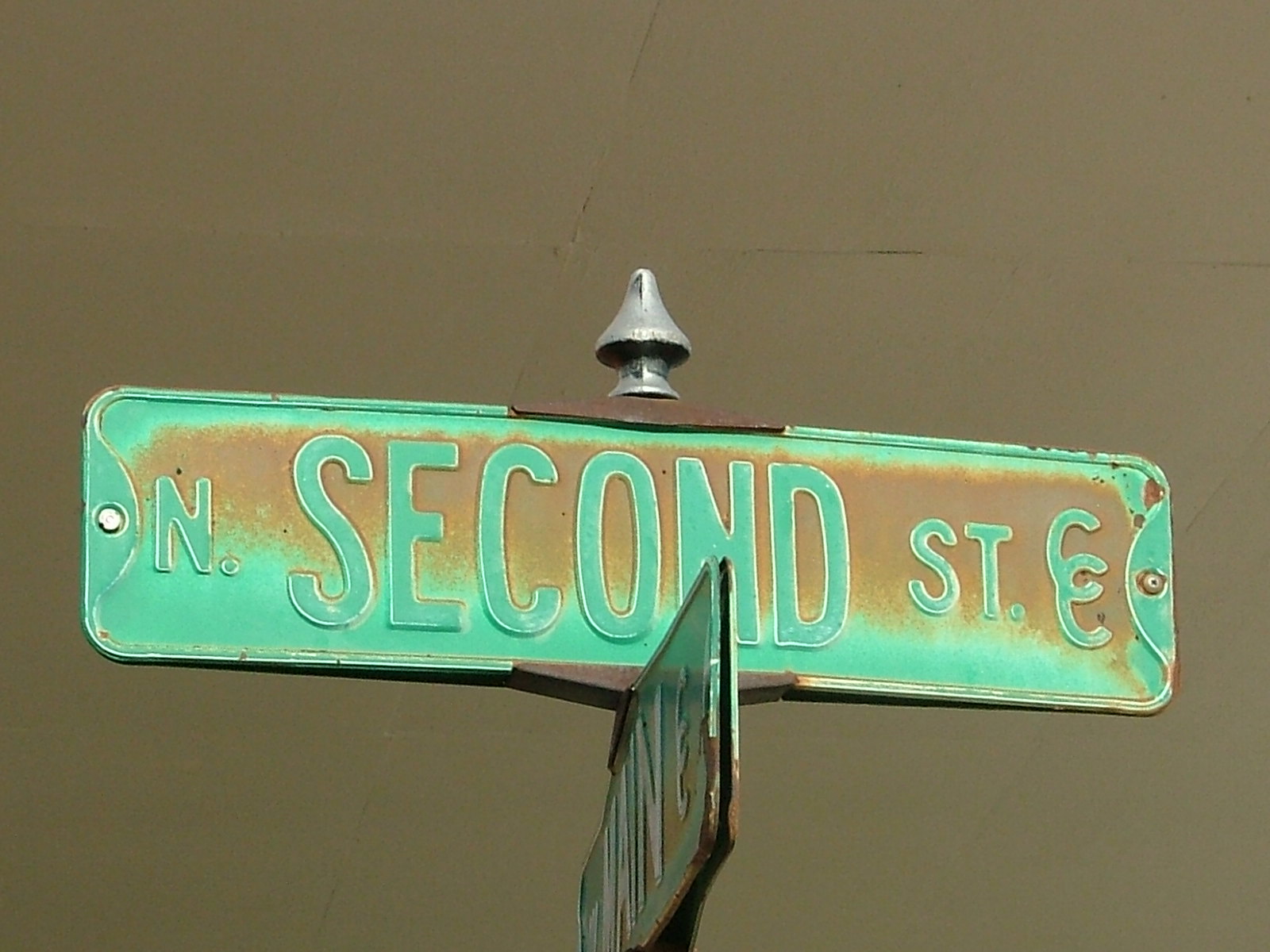A digitally animated depiction of a street sign with a unique, surreal lighting effect and highly realistic detailing that still falls short of photographic quality. The backdrop is a muted grayish-brown, adding to the overall somber tone of the image. The focal street sign, shaped as a rounded rectangle, prominently displays "North 2nd Street" with letters that appear embossed, adding depth to the text. The sign itself bears a rustic, weathered look with patches of brown and green rust, enhancing its aged appearance. Topping the sign is a distinct silver point. Beneath it, there's another sign that intersects perpendicularly, offering a multi-layered visual composition.